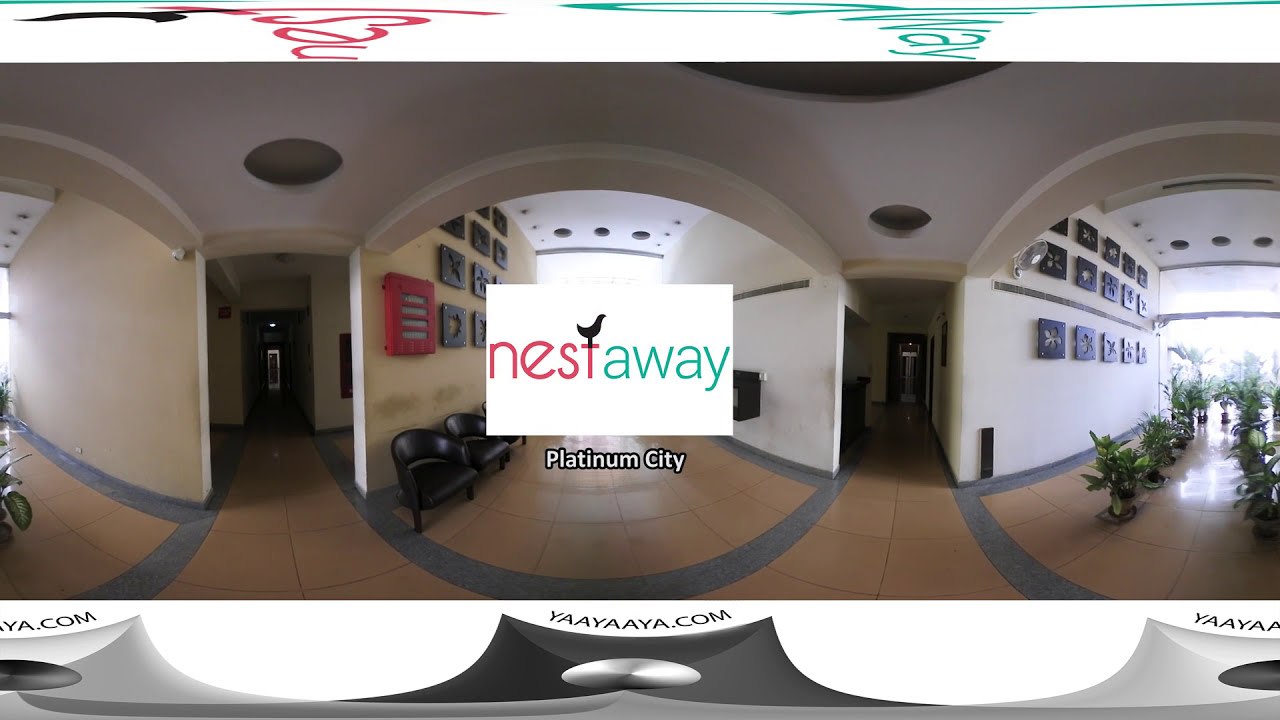The image showcases a panoramic view, likely of an office building entrance, with a fisheye lens effect causing some distortion. At the center of the image, a prominent white rectangle displays "Nest Away" with "Nest" in red, "away" in green, and a small black bird resting on the "T". Below, it reads "Platinum City". 

Towards the bottom, the text "Y-A-A-Y-A-A-Y-A dot com" is visible, accompanied by a silver sphere beneath it. The entrance hallway features white walls adorned with various plaques or decorations on the left side, including squares for decoration and a yellow wall with a red box outlining it. 

To the right, a pathway lined with rows of small potted plants is visible, leading towards a black door with a silver handle. The hallway also contains black seating reminiscent of a waiting area and brown and gray striped tiles. On either side of the image are contrasting ridges: white with black circles on the left and right, and a black ridge with a silver circle in the center. Clear glass doors can be observed towards the back of the hallway.